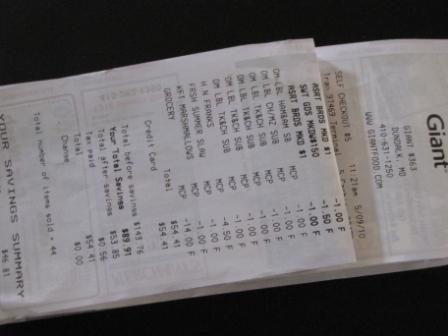The photograph depicts a low-resolution image of a long receipt from a Giant store, placed horizontally on a black surface. The picture has a slightly blurred, low-light quality, making some details difficult to read without turning the head sideways. The receipt is folded in thirds, obscuring parts of the text, and it prominently displays the store's logo "Giant" at the top, followed by the store's address, phone number, and website URL "giantfood.com". The image shows several purchases predominantly consisting of various types of meat subs and hot dogs, along with savings and totals. Despite spending $143 originally, the shopper saved $89 through discounts and coupons, reducing the total amount paid to $54. Shadows from the folds of the receipt are visible against the black background.